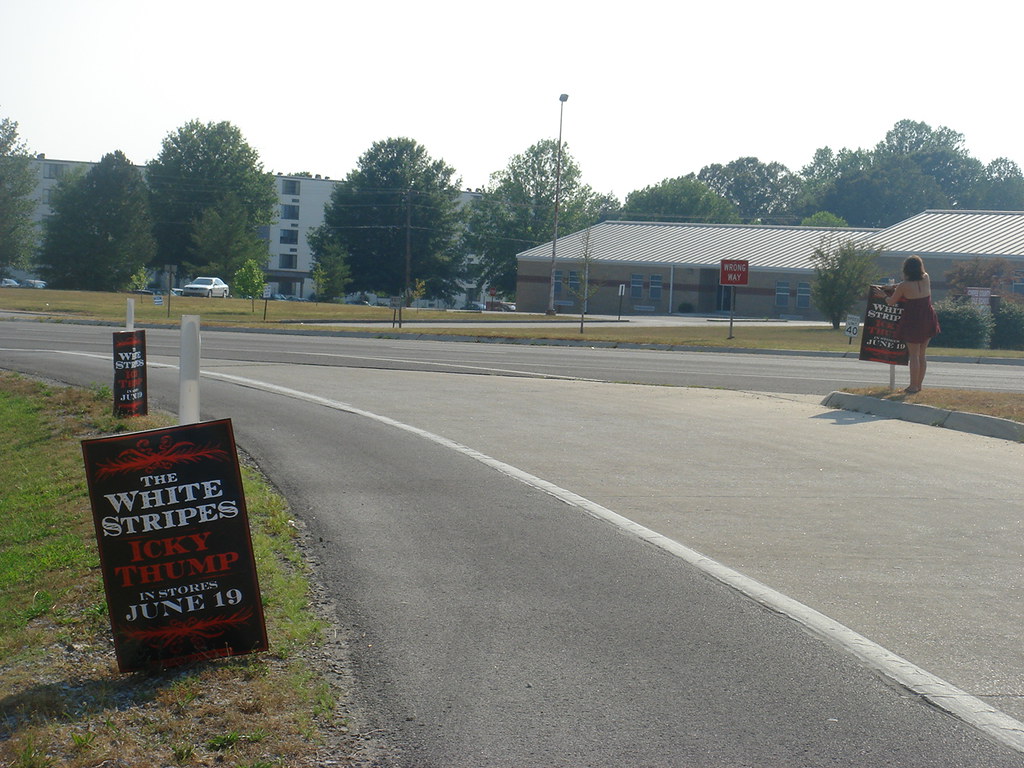This outdoor photograph captures a curved road that bends to the left and merges with another road in the background. The scene appears to be a suburban area with newly developed surroundings, evidenced by the small trees with support sticks. There are no vehicles on the road, which features a white line painted along its edge. Prominently, the image showcases a series of black placards with white and red text reading, "The White Stripes, Icky Thump, In Stores June 19th," indicating the photo is over a decade old. In the foreground, a placard is mounted on a white reflective post, and similar signs are visible further down the road. On the right side of the image, a woman in a maroon shoulderless sundress is mounting another placard to a reflective post, standing on a small traffic island. The sky overhead is overcast, and in the distance, there are two buildings with metal roofs—one resembling a hotel or apartment building and the other potentially a city building.